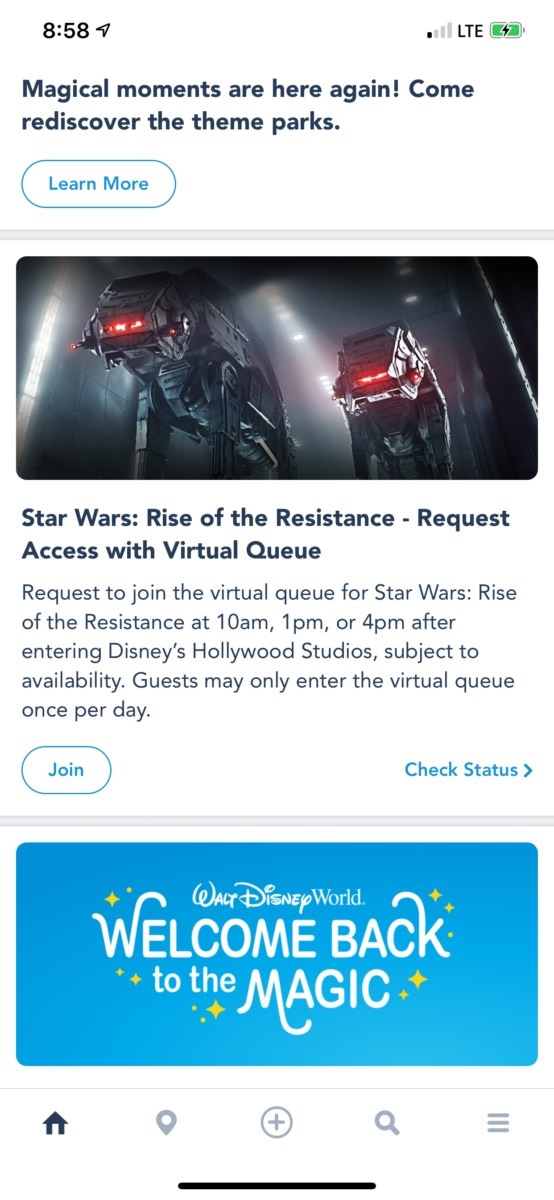### Descriptive Caption:

**Category: Websites**

The image displays a smartphone screen with the time showing 8:58, though it's unclear whether it's AM or PM. The screen shows an LTE connectivity icon and a fully charged battery. In navy blue text, it reads, "Magical moments are here again. Come rediscover the theme parks." Below this message is a button labeled "Learn More." 

There is a gray divider line, followed by an image depicting robotic figures from Star Wars. Accompanying this image, the text states: "Star Wars: Rise of the Resistance. Request access with virtual queue. Request to join the virtual queue for Star Wars: Rise of the Resistance at 10am, 1pm, or 4pm after entering Disney's Hollywood Studios. Subject to availability. Guests may only enter the virtual queue once per day." Beneath this information, there are options to "Join" or "Check Status."

Another gray line separates this section from the next. Below it, the text "Walt Disney World" appears, accompanied by "Welcome back to the magic" set against a blue background adorned with little stars. At the bottom of the screen are five icons: a house icon, a map icon, a plus icon, a search icon, and a menu icon.